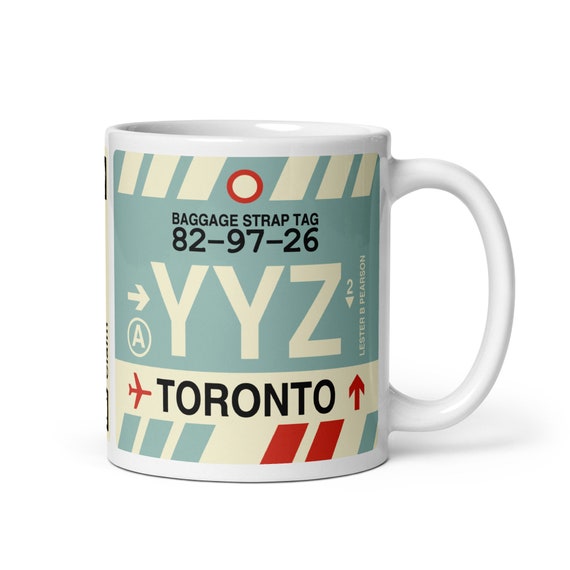This square product photo features a white ceramic coffee mug set against a pristine white background, casting a subtle gray shadow beneath it. The mug's handle is positioned on the right side, and it bears a retro-modernist design on its exterior. Dominating the mug's surface is a rectangular painting with curved corners, predominantly in a light turquoise hue. The top section features light yellow diagonals and is labeled with black text reading "baggage strap tag 82-97-26." Prominently displayed in large yellow letters is the airport code "YYZ." Below this, a light yellow band contains black capital letters spelling "Toronto," flanked by a small red airplane on the left and a red upward-pointing arrow on the right. This band sits atop a lower section of the painting that includes a mix of light green and red diamond shapes.